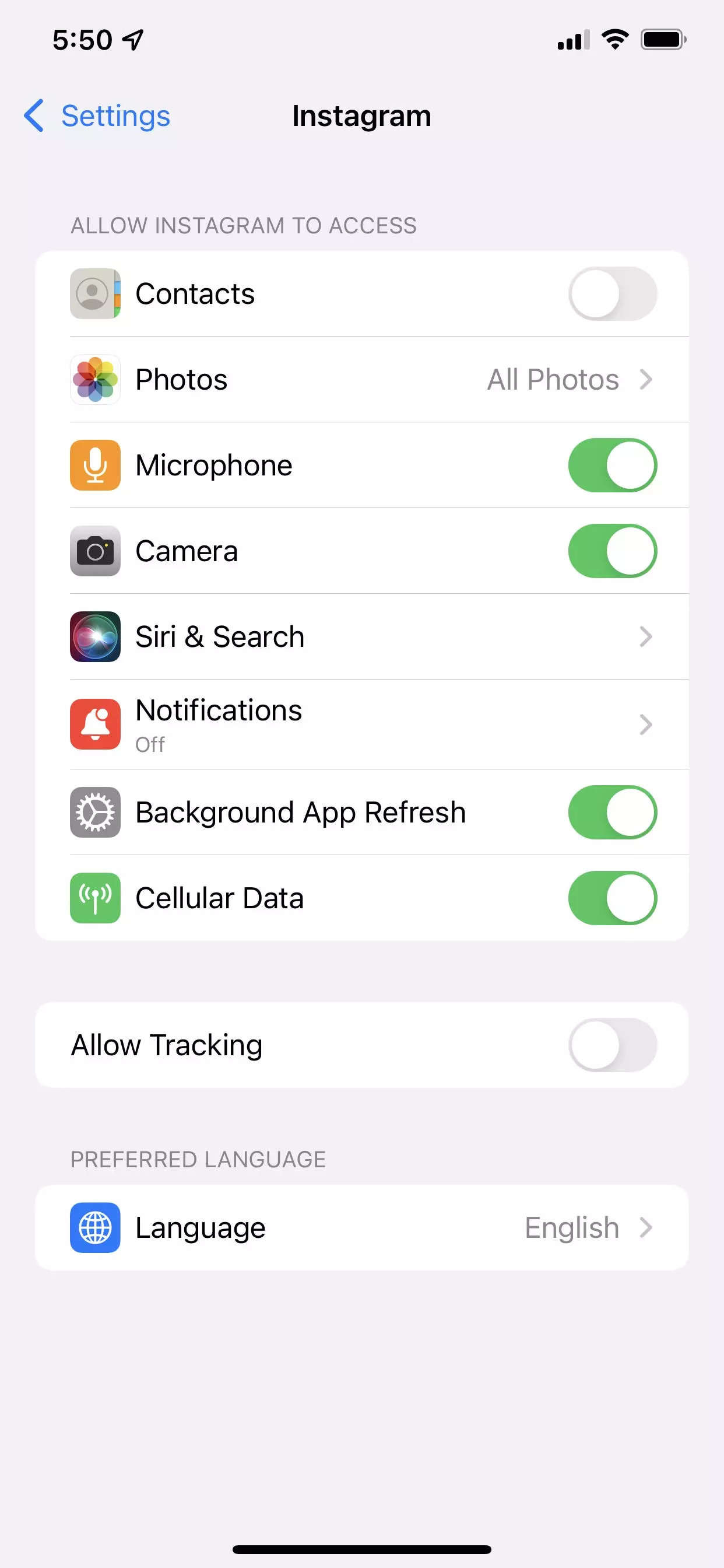Here is a cleaned-up and detailed caption for the image:

"The screenshot displays the settings for the Instagram app on a smartphone. At the top of the screen, there are options for Wi-Fi, Data, and Battery, followed by settings for allowing Instagram to access various features. The interface includes toggles, with selections such as 'Photos,' 'All Photos,' 'Microphone,' 'Camera,' and 'Siri & Search,' many of which are turned on, indicated by a green toggle. There are arrows next to 'Notifications' and 'Background App Refresh,' where Notifications are turned off and Background App Refresh is enabled. Additionally, the 'Cellular Data' and 'Allow Tracking' options both have green toggles, indicating they are active. The 'Language' is set to English, and a black line is visible at the bottom of the screen, separating these settings from additional options."